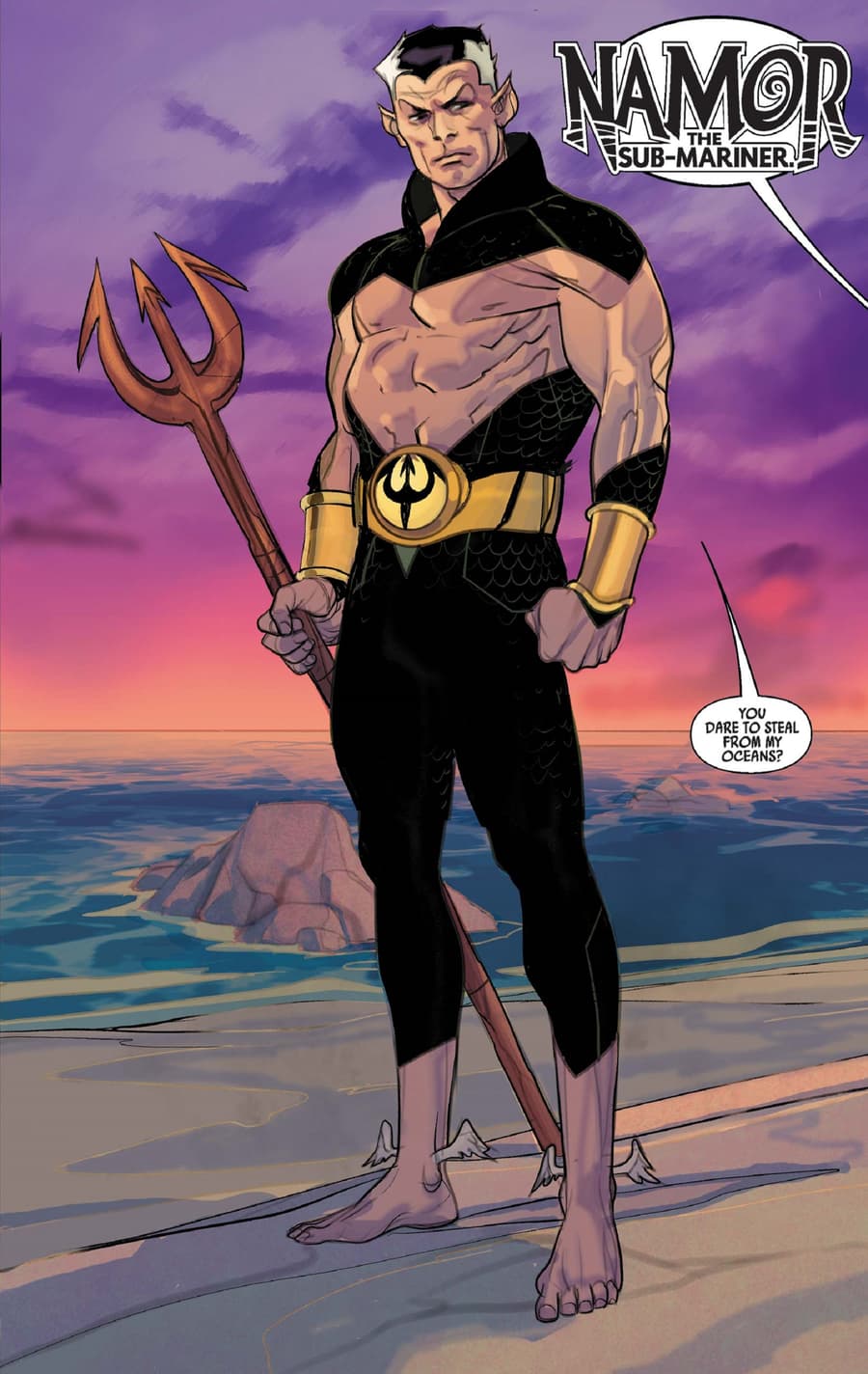This detailed comic book panel features Namor the Sub-Mariner, identifiable by the label in the top right corner and a speech bubble mid-page that reads, "You dare to steal from my oceans?" Against a backdrop of a purplish-reddish sunset over the ocean, with a large rock formation, Namor stands on the sandy shore. Namor is depicted as a muscular figure with predominantly black hair that has silver streaks on the sides, and characteristic pointed ears. He's wearing a black shroud draped over his shoulders and fastened at the neck, leaving his chest and abs exposed. His outfit includes black capri-length pants, golden gauntlets lined with black fabric, and a prominent gold belt with a large buckle featuring a yellow graphic. He wields a trident, reminiscent of a devil's trident, and has small wings on his ankles that enable flight. Namor's overall appearance emphasizes his regal and formidable presence as a guardian of the ocean.